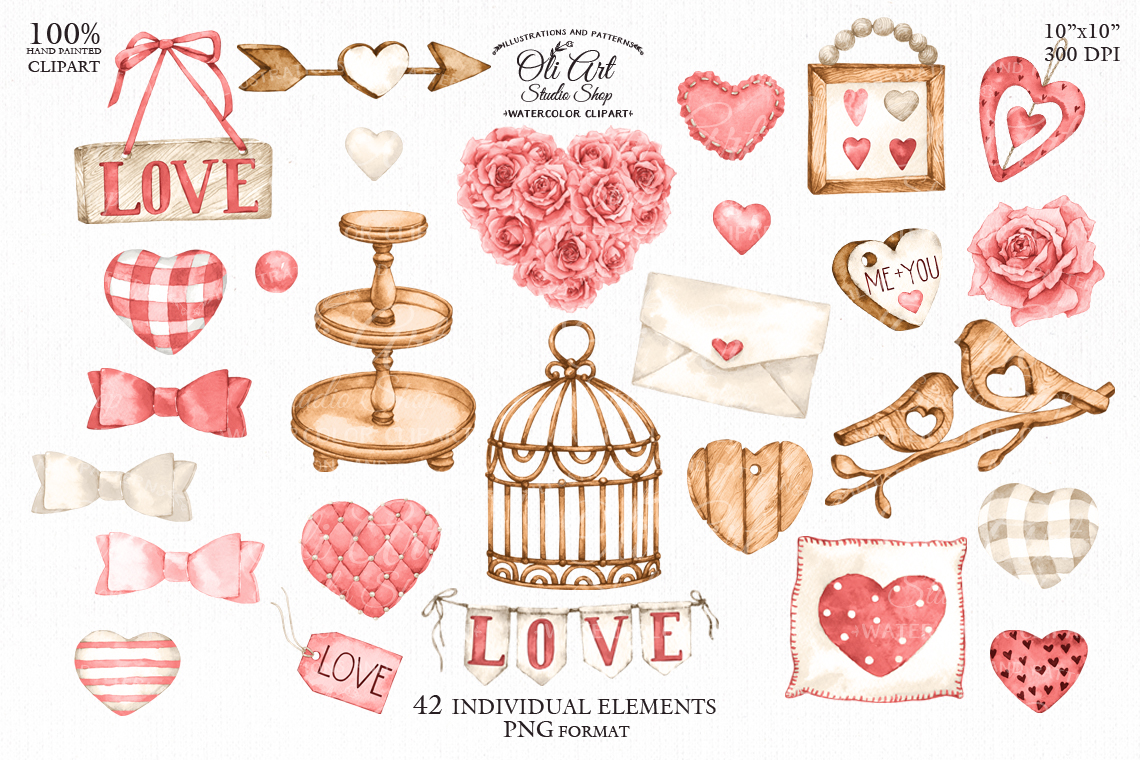This image is a collage of 42 hand-painted watercolor clip art elements from Ollie Art Studio Shop, arranged in a horizontal rectangle without borders. The collection features a variety of elements primarily in shades of pink, white, and gold. At the top left, black text reads "100% hand-painted clip art," and in the center top it states "Ollie Art Studio Shop watercolor clip art." The top right notes the dimensions "10 by 10 inches, 300 DPI," while the bottom center specifies "42 individual elements PNG format."

The elements within the collage include multiple hearts in various designs such as checkered, striped, and plaid patterns, and a pink and white polka dot heart. Some hearts bear messages like "me and you." There are also ribbons tied into bows in pink, red, gold, and white, alongside squares and rectangular blocks with pink letters spelling out "LOVE." Additional objects include a three-tiered gold stand, a gold arrow with a white heart, a gold bird cage, and a brown frame with a pearl hook containing four hearts. A white pillow, a white envelope with a pink stamp, various pink flowers, and two doves with heart cut-outs further enhance the love-themed collection.